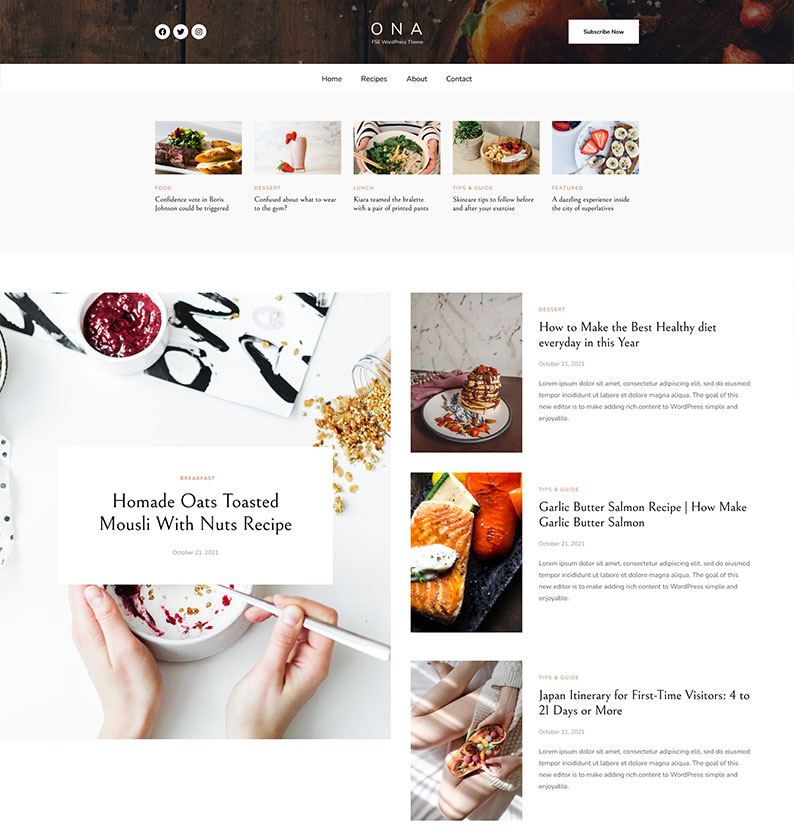**Screenshot Description: Detailed Website Layout**

The screenshot showcases a colorful, aesthetically pleasing website layout. 

**Header Section:**
At the very top, a dark, multi-colored bar stretches across the screen, featuring "ONA" in prominent white lettering. Below "ONA," there is additional white text, but it is too small to be legible. On the left side of this bar, three white circles contain social media icons: Facebook, Twitter, and Instagram, in that order. To the upper right, still on the multicolored bar, a white button with "Subscribe Now" written in black is visible. 

**Navigation Menu:**
Directly beneath the top bar, the navigation menu displays four labels in black text: "Home," "Recipes," "About," and "Contact."

**Main Content Area:**
1. **Thumbnail Image Row:**
   - **First Thumbnail:** A somewhat unclear image that looks like a piece of meatloaf topped with a Reuben sandwich. The description is blurry and unreadable.
   - **Second Thumbnail:** A glass of strawberry shake adorned with strawberries both inside the glass and attached to its rim.
   - **Third Thumbnail:** A white salad bowl, possibly containing chopsticks, held by someone in a white and black striped sweater.
   - **Fourth Thumbnail:** Difficult to discern due to blurriness, likely contains contents in a wooden bowl.
   - **Fifth Thumbnail:** A white plate with slices of banana on the right and slices of strawberry on the left, arranged with a spoon at the 8 o'clock position.

2. **Feature Section:**
   - **Larger Image:** Located at the bottom left corner, it showcases a detailed caption in a white window stating "Homemade Oats Toasted Muesli with Nuts Recipe." Visible are a couple of white ramekin dishes, with hands stirring contents in a white ramekin dish using a chopstick.

3. **Vertical Image Sidebar:**
   - **Top Image:** Picture of a popover-like dish on a plate with the text "How to Make the Best Healthy Diet Every Day This Year."
   - **Middle Image:** Displays a piece of salmon with the caption "Garlic Butter Salmon Recipe: How to Make Garlic Butter Salmon."
   - **Bottom Image:** Reveals someone’s bare legs holding a fruit bowl, captioned "Japan Itinerary for First-Time Visitors: 4 to 21 Days or More."

The design is cluttered with images and text, some of which are too blurry to decipher, yet it effectively conveys a rich, appetizing spread of content focused on recipes and lifestyle tips.